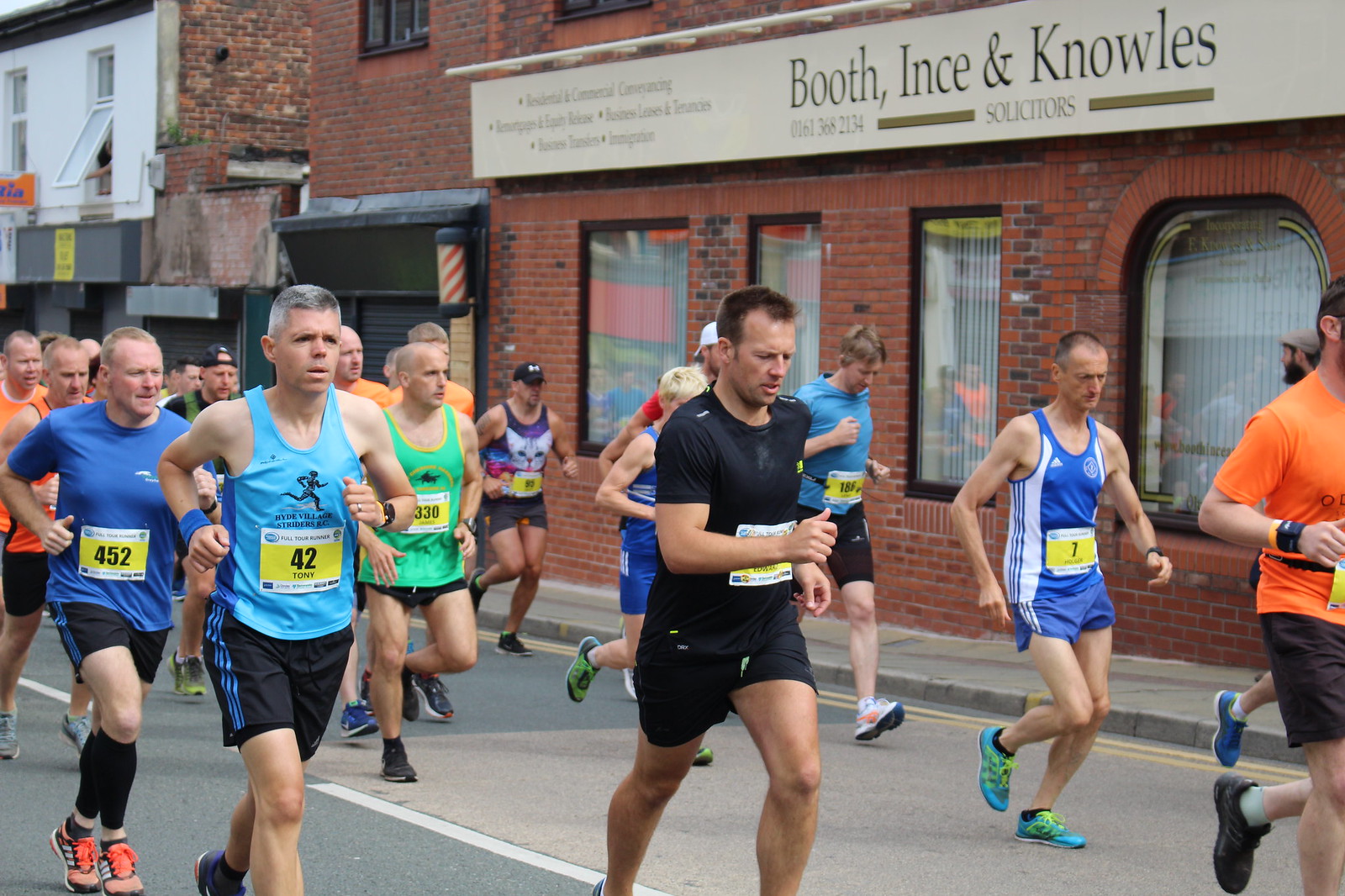This image captures a marathon taking place on a quaint downtown street lined with red-brick buildings. The focal point is a runner at the center wearing a black shirt and black shorts, his face tilted slightly downward in concentration. To his left, a man in a blue tank top with a running silhouette emblem is prominent, sporting a race bib numbered 42 with a white and yellow background. This runner has black shorts accented with blue stripes. The diverse group of runners includes men of various ages, from their 40s to their 60s, all clad in different styles of running attire, predominantly shorts and tennis shoes.

The street scene behind the runners features a mix of well-maintained and slightly rundown buildings, adding to the charming, somewhat gentrified feel of the area. Standing out in the background is a brick building with windows outlined in black, topped by a sign that reads "Booth, Eats, and Knowles. Solicitors." Further back, a white building with a partially open window reveals a person pushing it open. Notably, an old-fashioned barber pole adds an element of nostalgia to the setting. This vibrant, lively marathon snapshot is enriched with the quaint details of its urban backdrop and the dedicated runners pushing through the course.